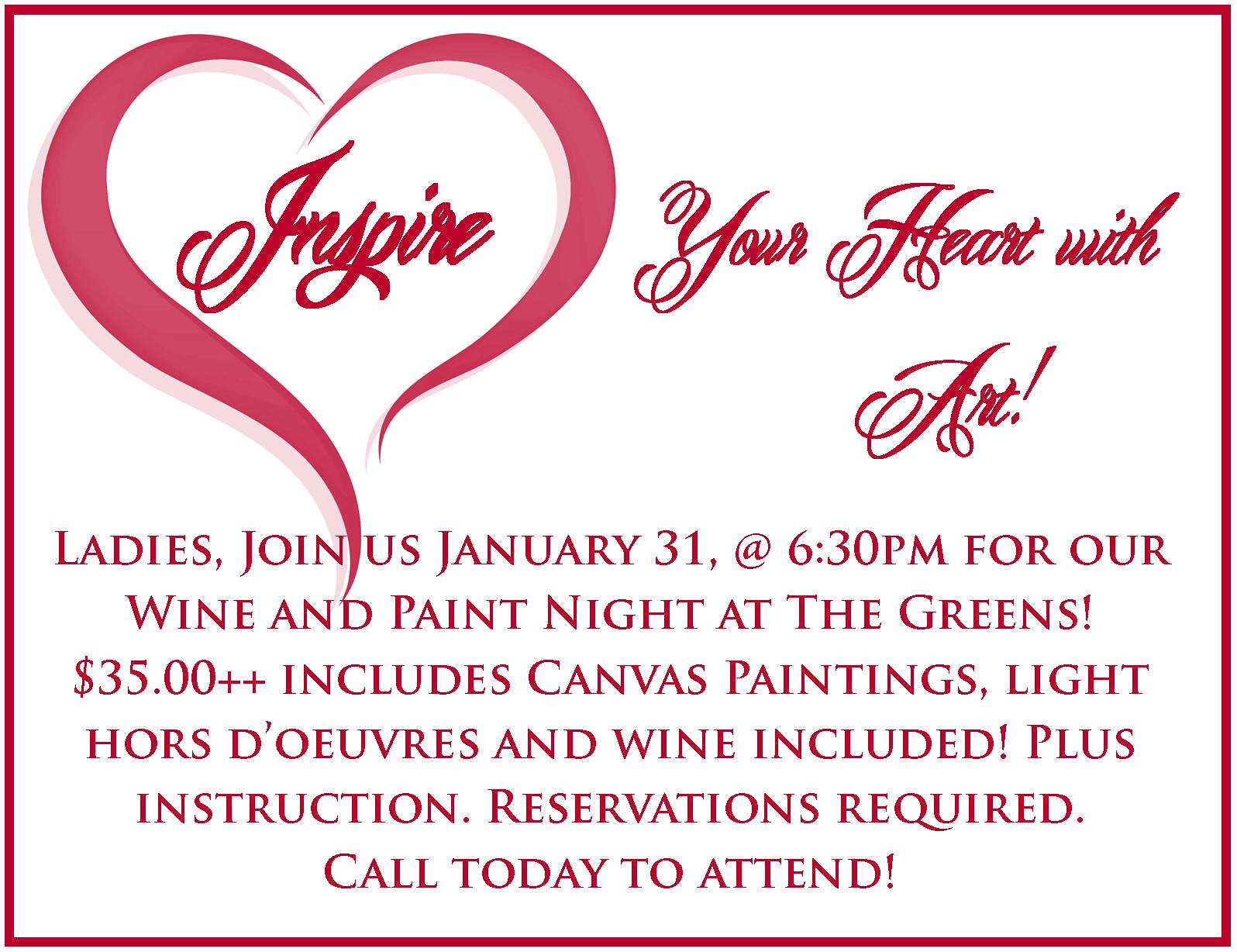The image features a square, large, rectangular design with a thin red border on a white background. In the top left corner, there is a pink heart with swirly details, and inside the heart, in cursive red writing, it says "Inspire." To the right of the heart, the text reads "your heart with art!" In bold red letters toward the bottom, the invitation is clear: "Ladies, join us on January 31st at 6:30 p.m. for our wine and paint night at The Greens. $35 includes canvas paintings, light hors d'oeuvres, wine, and instruction. Reservations required. Call today to attend!" The poster exudes a cozy, festive invitation for a wine and paint event aimed specifically at ladies.